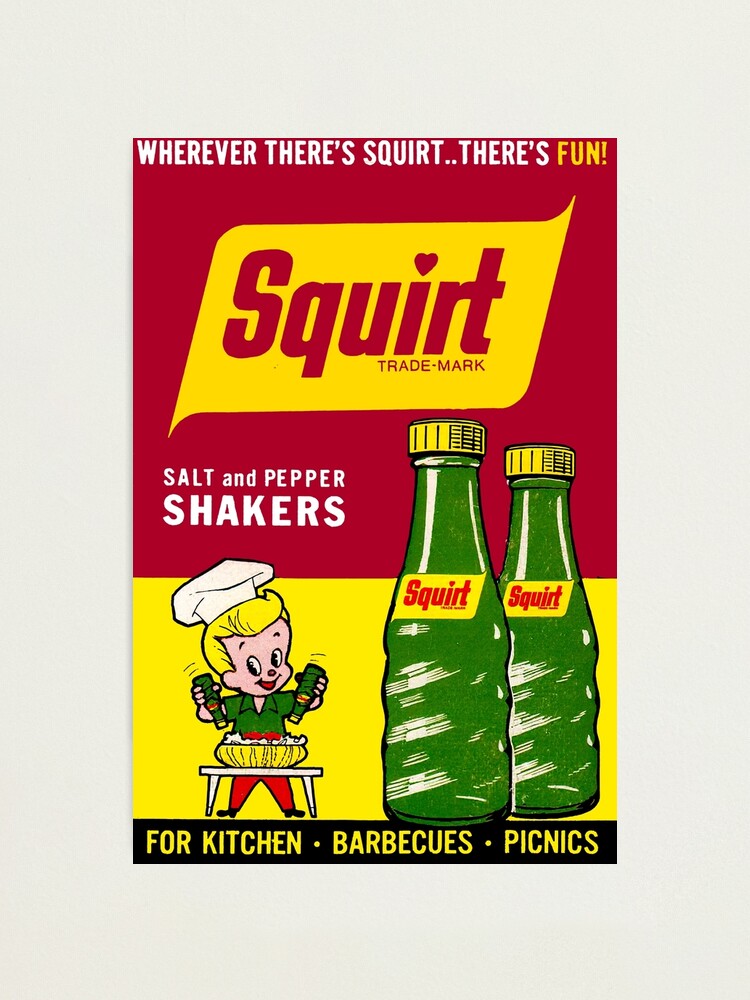This advertisement for Squirt features a nostalgic, colorful design reminiscent of vintage product packaging. The top half has a vibrant orange-red background with the slogan, "Wherever there's Squirt, there's fun!" prominently displayed in white and yellow text. The word "fun" and the exclamation point are highlighted in yellow. Below is the Squirt logo, presented in a unique rounded-corner trapezoidal shape pointing outwards at the top right and bottom left. The logo text is red, with the "i" in "Squirt" dotted by a heart, and a small "trademark" indication beneath it.

On the bottom left of the red area, "salt and pepper shakers" is written in small white text. The main visual features two green Squirt bottles with yellow caps; these bottles extend from the yellow lower half into the red upper half. To the right, a cheerful illustration shows a blonde-haired boy in a chef's hat, green shirt, and red pants, shaking the bottles over a bowl of food.

The design is anchored by a black bar at the very bottom, with yellow text that reads, "For Kitchen, Barbecues, Picnics," adding a functional touch to the playful imagery.